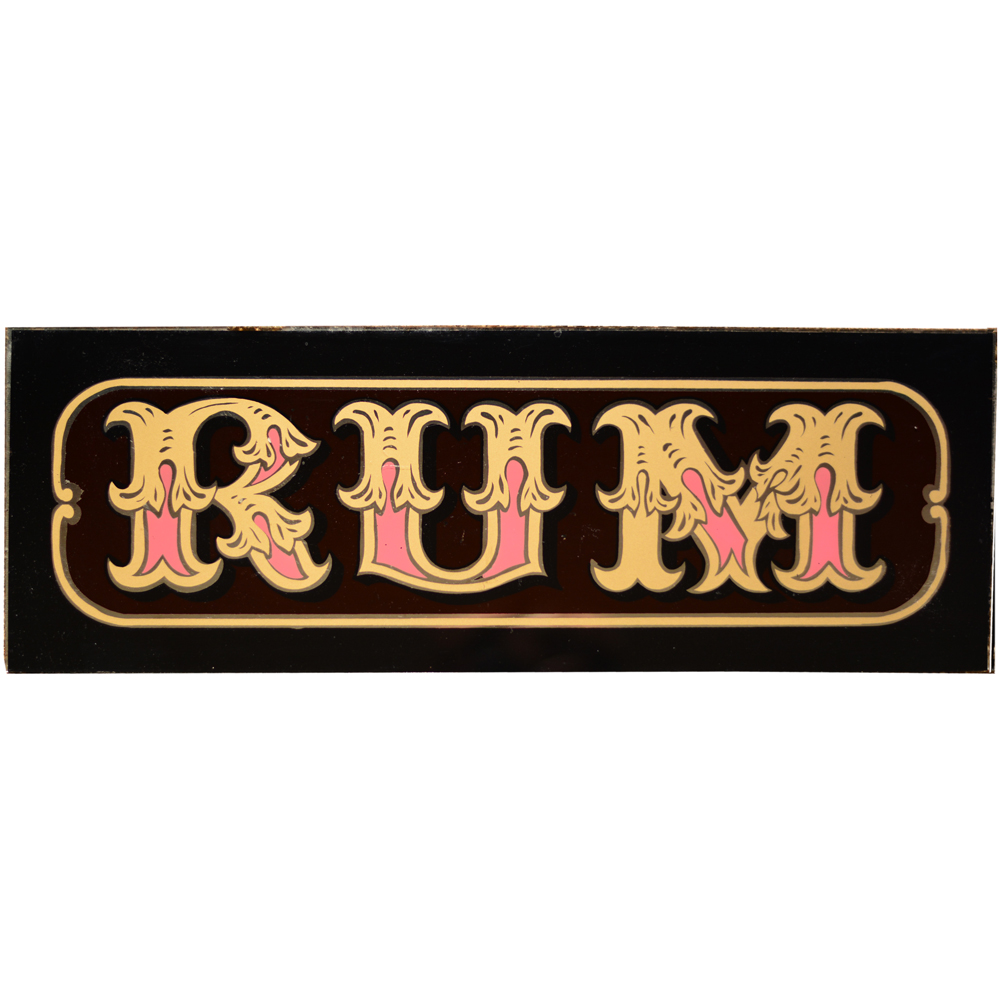The image showcases a black, rectangular label with a gold scroll border that has rounded edges. This ornate label prominently features the word "RUM" in a sophisticated filigree font, which evokes a vintage Western saloon sign. The word "RUM" is two-toned: the upper half of each letter is a deep gold, while the bottom half is pink. The text is elegantly detailed, with the gold outlines adding to its intricate appearance. Despite slight variations in descriptions, all three captions agree on the black background, the gold and pink coloration of the text, and the opulent styling of the font, creating a visually striking and elaborate design.